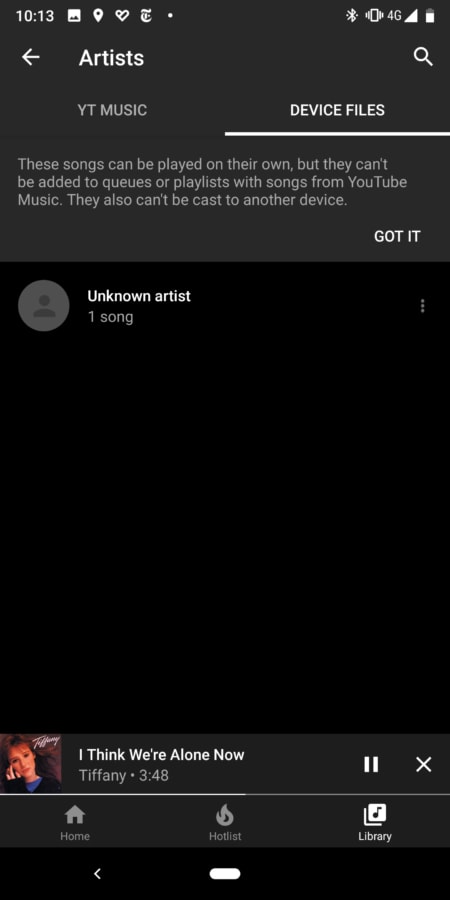This is a screenshot of the "Artist" tab on the YouTube app, viewed on a mobile phone set to night mode with a black background. At the top left corner of the screen, the status bar displays the current time, an image icon, a location icon, a New York Times icon, and a heart icon. On the right side of the status bar, there are icons indicating that Bluetooth is enabled, the phone is set to vibrate mode, 4G network connectivity, signal strength, and battery level.

Just below the status bar, the header reads "Artists" with a left-pointing arrow on the left side and a magnifying glass icon (for search) on the right side. Under this header is a dark box with a slightly lighter top segment featuring two tabs: "YouTube Music" and "Device Files," with "Device Files" being the selected option. The box contains a description and a "Got it" button in the bottom right corner.

Below this section, "Unknown Artist" is listed alongside one song, with a blank profile picture to the right and a three-dot action menu icon further to the right. At the bottom of the screen, the currently playing song is "I Think We're Alone Now" by Tiffany. The album thumbnail is displayed on the left, along with pause and exit icons to the right of the song title. Finally, the bottom navigation bar shows three options: "Home," "Hotlist," and "Library."